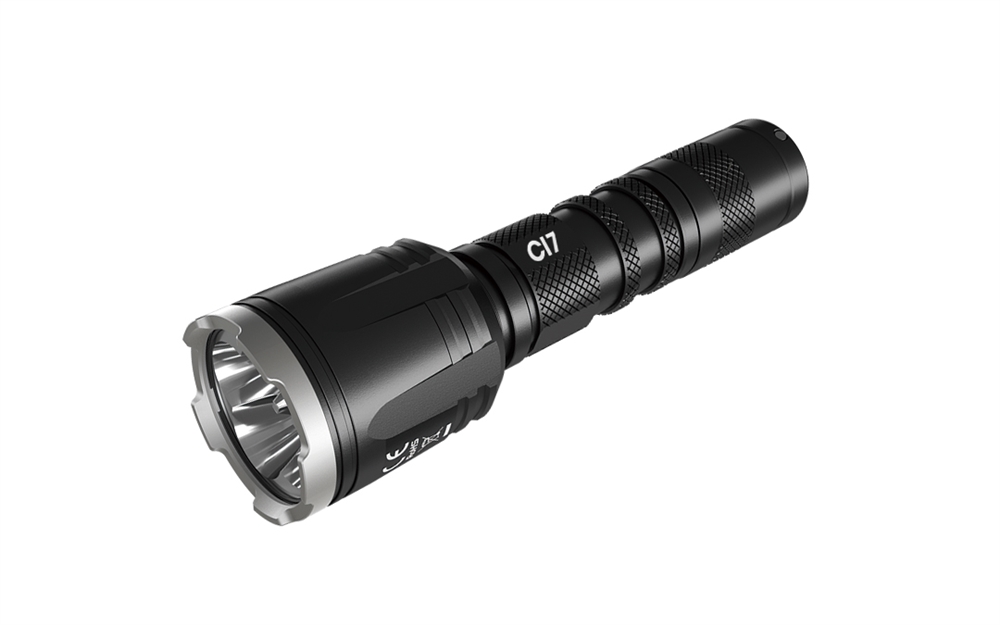The image depicts a robust, military-grade black flashlight with a muted finish to minimize reflections. The flashlight features a textured grip with ridges designed for secure handling. The handle appears adjustable, possibly telescoping to extend its length. Notably, the head of the flashlight is larger and constructed from a solid, sturdy metal, distinguished by a light silver band around the edge. Near the head, there is some unreadable writing tilted to the side. The side of the flashlight bears the white text "C17." Additionally, the image captures the bulb at the tip of the flashlight, situated in the lower left of the picture, with the handle extending towards the upper right.